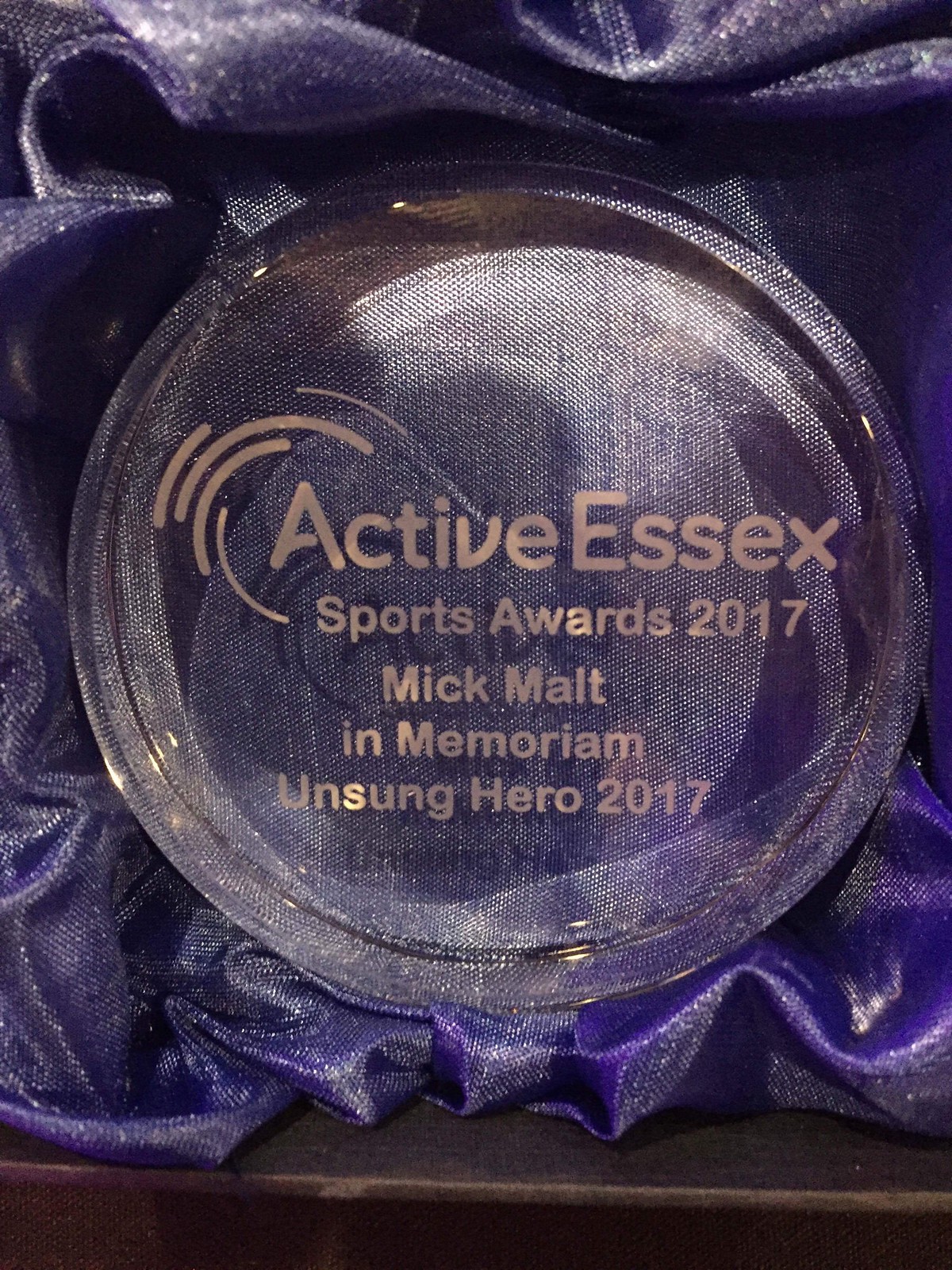The image is a photograph of a clear, circular crystal object, possibly a trophy or a decorative item, labeled with "Active Essex Sports Awards 2017, Mick Malt, In Memoriam, Unsung Hero 2017" in a bronze or gold font. This crystal piece is placed inside a brown wooden box, nestled in a luxurious, velvety fabric that appears to be purple with a shimmer of gold or silver flecks. The fabric surrounds the crystal object, providing a rich, ornate background. Additionally, there is a bright light overhead, reflected in the crystal surface, adding to the object's overall shimmery and elegant appearance.